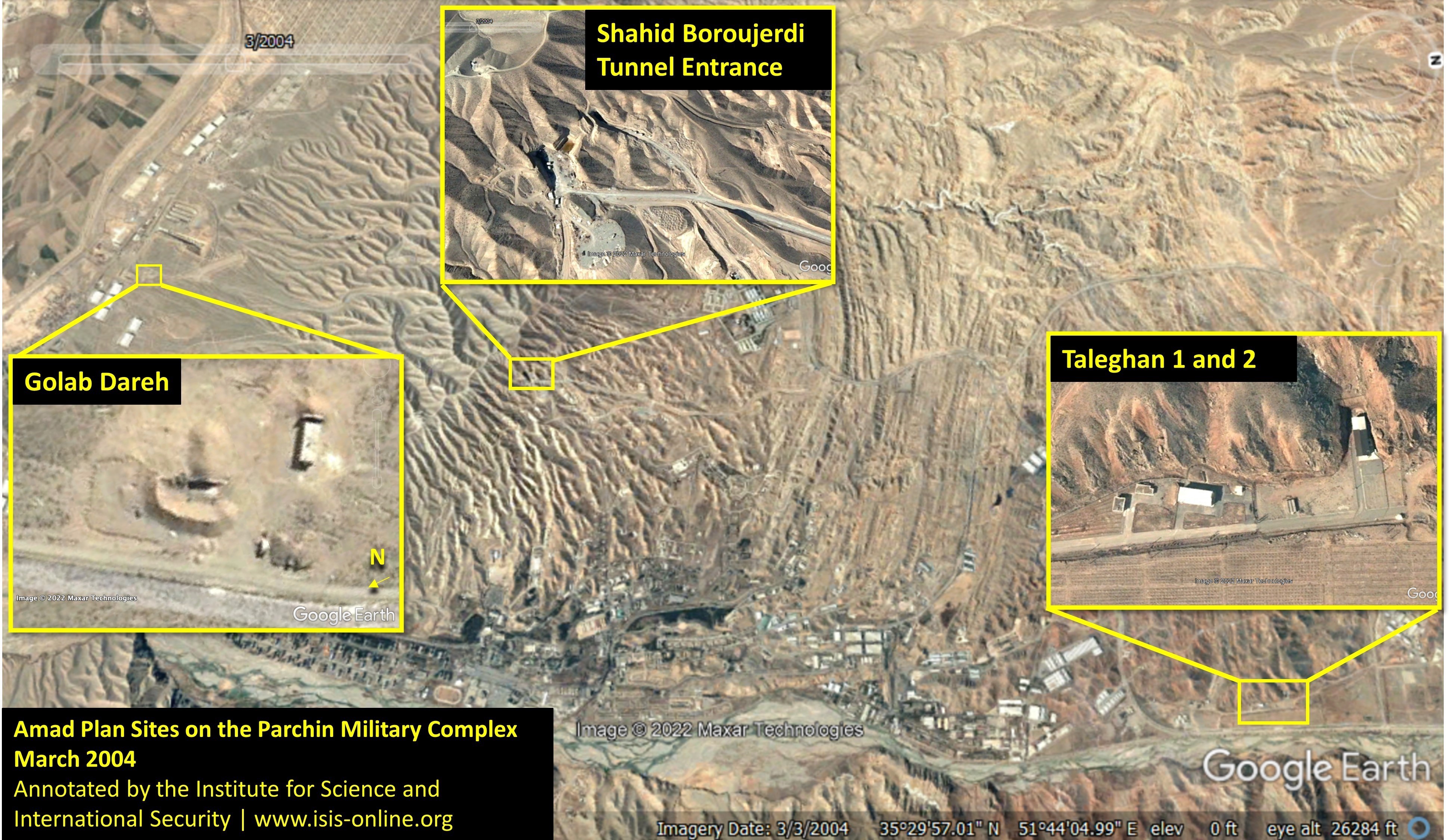This is a detailed Google Earth satellite image dated March 3, 2004, depicting a desert-like terrain with various highlighted areas. The overall landscape is characterized by reddish-tan dirt, rocky formations, and striations indicative of land elevations. Three significant locations are marked with yellow rectangular boxes. At the top, text reads "Shaheed Boroujerdeh Tunnel Entrance," highlighting a road and possible tunnel entrance. To the left center, another yellow box is labeled "Golab Daray," focusing on a landmass feature. On the right, another marked area says "Taleghan 1 and 2," likely pointing out additional infrastructure or tunnel entrances. At the bottom left, within a black-bordered label with yellow text, information states "Amad Plan Sites on the Parchin Military Complex, March 2004, annotated by the Institute for Science and International Security, www.isis-online.org." The bottom right corner of the image contains white text indicating the source and date: "Google Earth, Imagery Date 3-3-2004," alongside specific longitude and latitude coordinates. This annotated image serves to highlight these key military or industrial sites within the Parchin Military Complex.